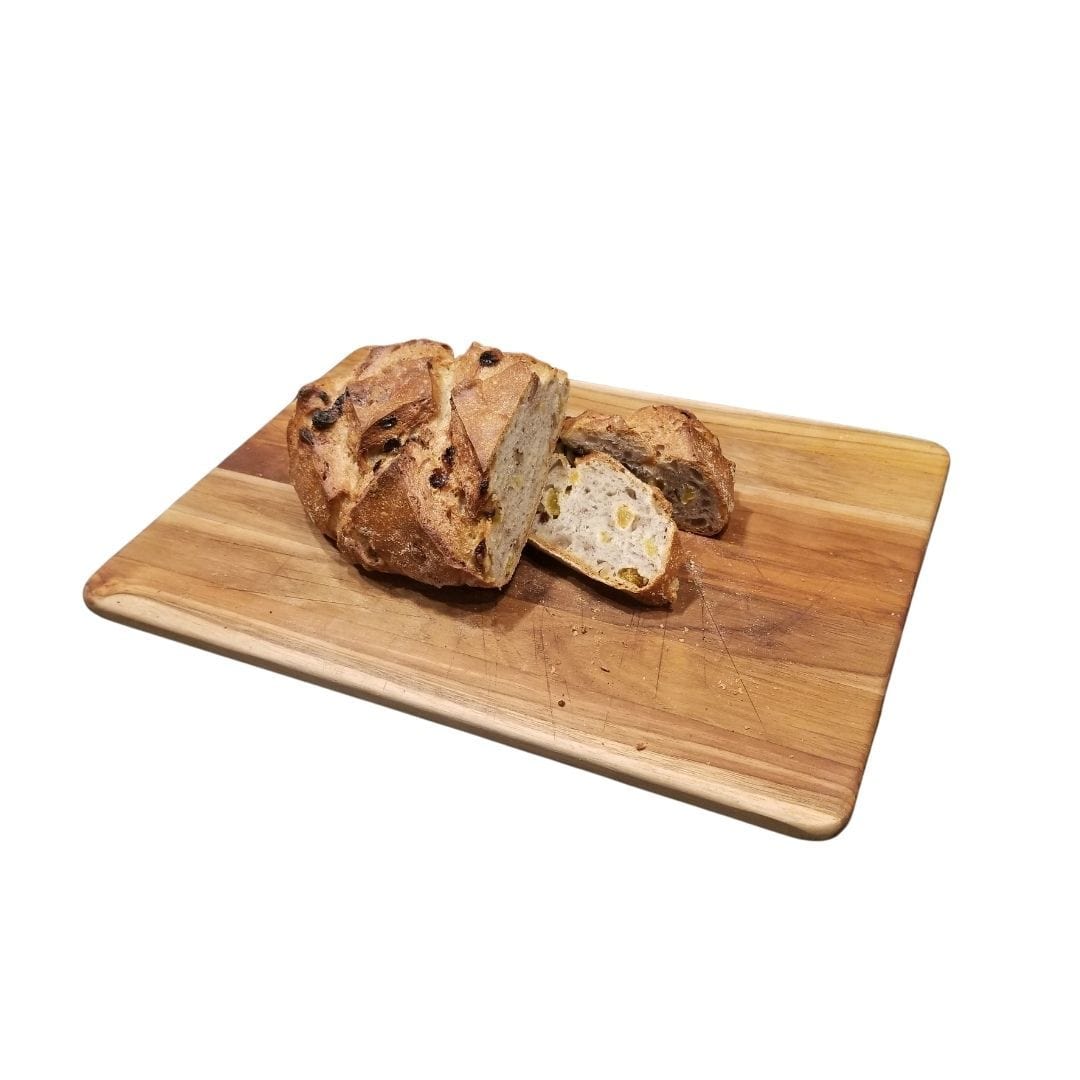In the photo, a beautifully crafted wooden cutting board with rounded edges and a mosaic of different brown shades showcases a rustic loaf of raisin bread. The bread, rich with a light brown crust, is partially sliced; the larger end piece is on the left, while two smaller slices are on the right. The golden-brown crusted exterior contrasts with the creamy interior, which features airy gaps giving it a slightly coarse yet inviting texture. The loaf reveals hints of raisins and a slight toasted touch on the crust. The background is a clean, stark white, emphasizing the warm, hearty colors of the bread and the wooden board. This inviting scene looks like an ideal setup for a delicious meal.